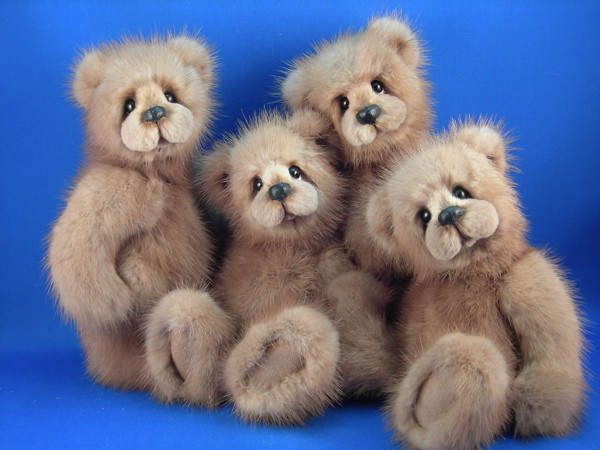In this color photo, four identical, light brown teddy bears are arranged against a bright blue background. Each teddy bear has a pinched face with small, beady brown eyes and a little brown nose. Their fur is notably fuzzy and thin, especially on their heads, giving a slightly bald appearance. The teddy bears are positioned tightly together, with two towards the bottom and two placed a bit higher, resembling a cozy, hugged-up group. Their tiny rounded ears, soft round jaws, fluffy arms, and feet contribute to their overall cute and slightly eerie look as they stare directly into the camera. One of the teddy bears appears to be slightly laid over, with another tenderly resting its head on it, adding to the sweet, endearing composition of the scene.